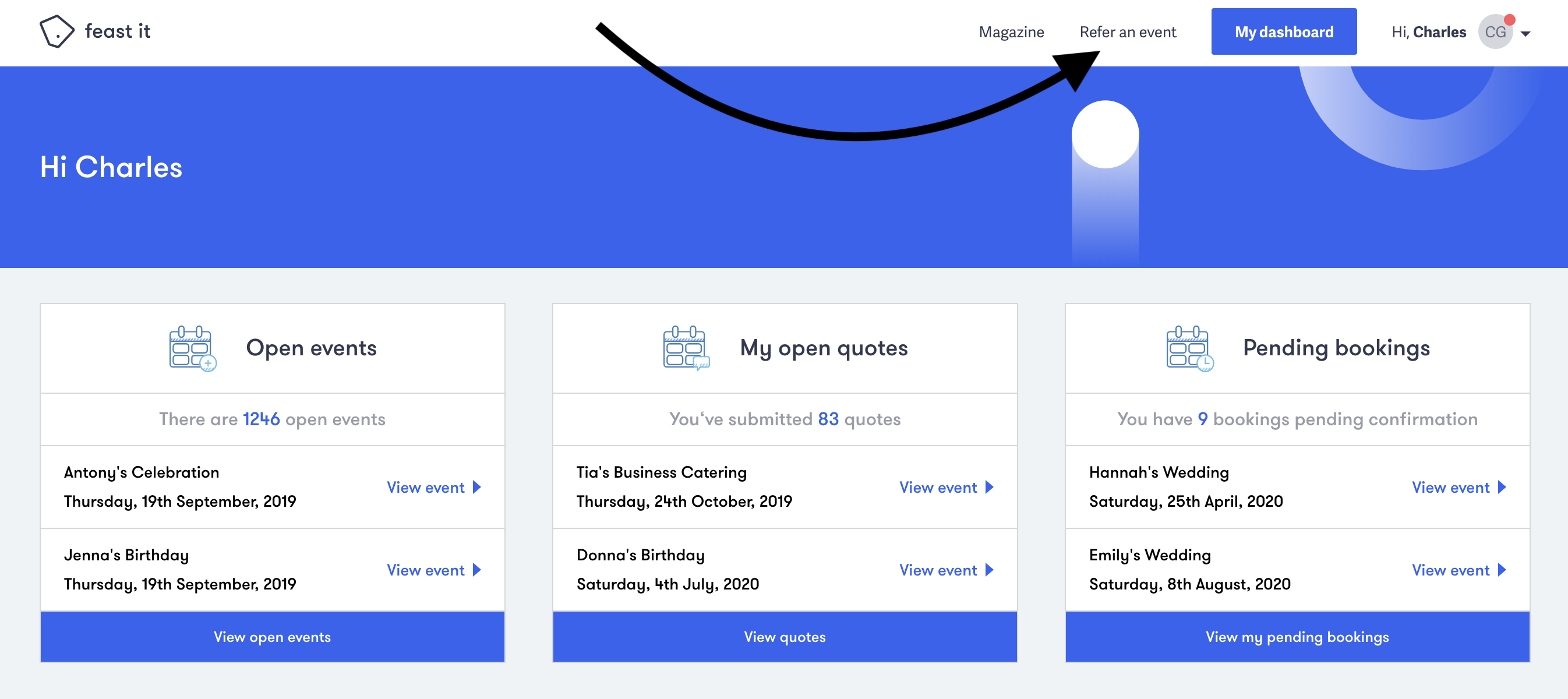The image appears to be a screenshot from a computer screen, displaying a dashboard interface. 

In the top left corner, there is an icon resembling a price tag, alongside the text "Feast It." To the far right, several options are visible, including "Magazine," "Refer an Event," and a blue "My Dashboard" button. The screen also greets the user with "Hi Charles," and includes a dropdown menu icon for accessing account settings.

A black arrow with a curved line points towards the "Refer an Event" option. The dashboard features a dark blue border on the left with another "Hi Charles" greeting. Towards the right, there is a white circle with a line underneath it, and in the upper right corner, a white semicircle.

Below, the interface transitions into a gray background divided into three main sections:

1. **Open Events**:
   - Displays a total of 1,246 open events.
   - Lists events such as "Anthony's Celebration" on Thursday, September 19, 2019, and "Jenna's Birthday" on the same date, each accompanied by a "View Event" link.
   - A blue bar labeled "View Open Events" is positioned beneath the event listings.

2. **My Open Quotes**:
   - Indicates that 83 quotes have been submitted.
   - Shows events like "Thea's Business Catering" and "Donna's Birthday" on Saturday, July 4, 2020, each with a corresponding "View Event" link.
   - A blue button marked "View Quotes" is situated below the quotes section.

3. **Pending Bookings**:
   - Notes that there are nine bookings pending confirmation.
   - Lists bookings such as "Hannah's Wedding" and "Emily's Wedding," each with a "View Event" link.
   - Below the listings, a prompt reads "View My Pending Bookings."

This detailed description captures the layout and specific elements visible on the dashboard interface in the image.